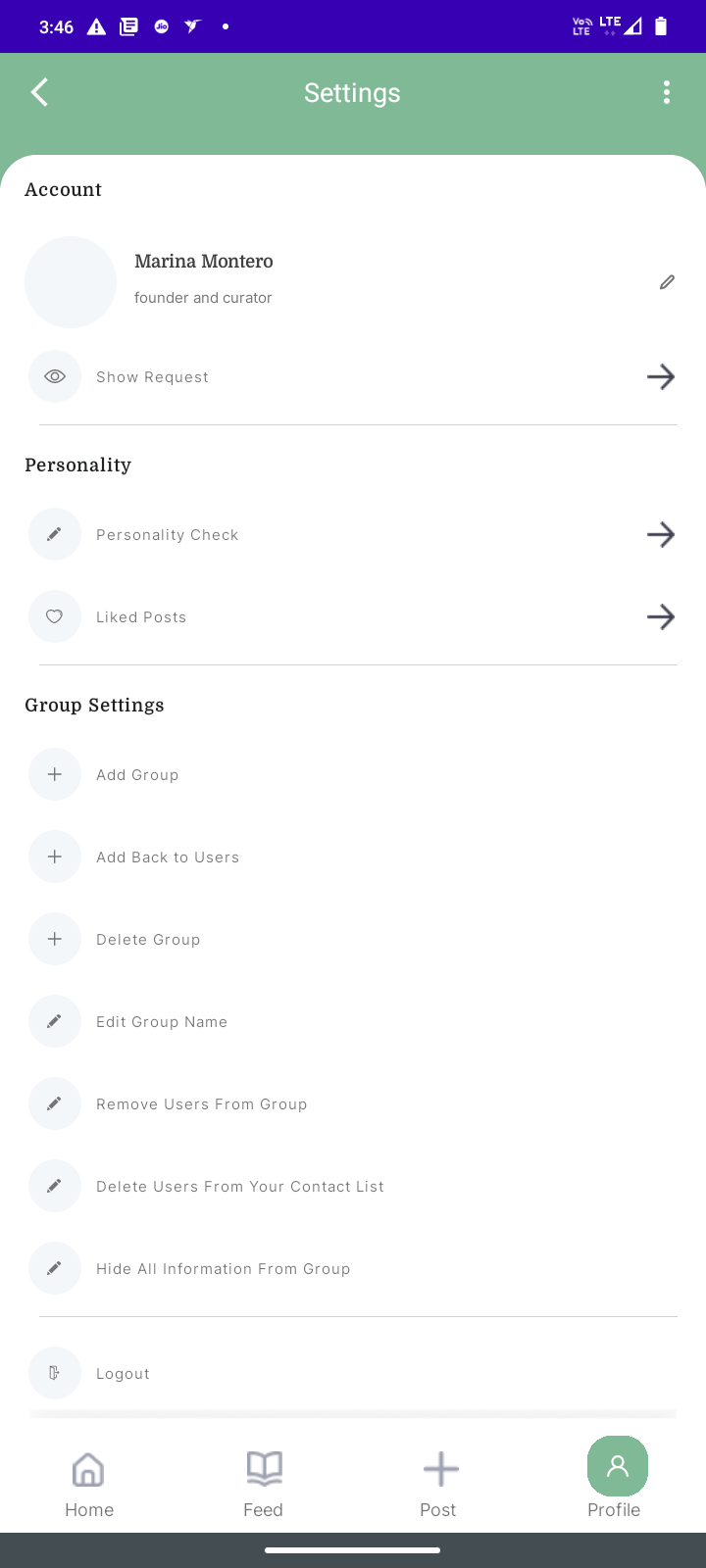The image depicts a user interface of a social media platform with various interactive elements and controls. At the top, there's a shout out to "346" highlighted, likely indicating a number of notifications or messages. Icons using a blue and green color scheme are prominently displayed, providing access to different settings and configurations. 

On the left side, there's an "LT" icon next to a green left arrow that leads to settings. Dotted lines separating sections indicate different account management options. The middle section shows account details with a white background. The user's name appears as "Ontario," labeled as the founder and creator, indicating their important role within the platform.

A section labeled "show request" suggests pending notifications or actions. Below it, several group management options are listed, including "add group," "delete group," "edit group name," "remove users from group," and options to manage user contacts such as "delete users from contact list" and "hide all information from group." 

At the bottom, there's a logout option and navigation buttons for home, feed, post, and profile. The background is predominantly white with blue and green highlights, ensuring that key interactive elements stand out. A white line runs through the middle, possibly dividing different sections or types of content on the interface. This detailed interface layout provides comprehensive tools for user and group management in a visually organized manner.